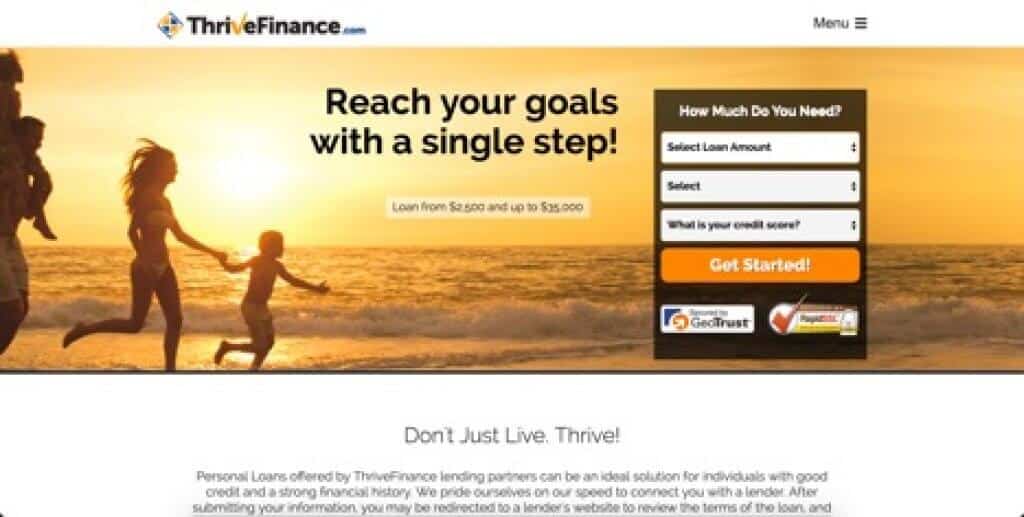Screenshot Description: Thrive Finance Website

At the top of the screenshot, the image is blurred, making the details difficult to discern. However, visible in this section is a logo in a diamond shape composed of two yellow triangles and two black triangles. The text "Thrive Finance" is present, with the 'V' stylized as a yellow check mark, while the remaining text is in black. To the right of the logo, it possibly says ".com," although this part remains too blurry to confirm. Further to the right, the word "Menu" is noticeable accompanied by a hamburger menu icon.

Below the blurred section, there is a hero image depicting a scenic family moment. A man carries a child on his shoulders, and to their side, a woman is running hand-in-hand with a younger boy. They are all near the ocean during sunset, contributing to a predominantly golden-tinted backdrop. The sky features subtle waves and gentle foam at the shore.

Overlaying this idyllic scene, in large black text, is the motivational phrase: "Reach your goals with a single step!" Beneath this text, in white, it states: "Loan from $2,500 and up to $25,000."

To the right, there is a rectangular section prompting user interaction with the question, "How much do you need?" This is followed by three drop-down options for selecting the loan amount and credit score. Accompanying these is a large, inviting orange button labeled "Get Started."

Further down the page, a GeoTrust icon is visible alongside another payment trust logo featuring a prominent red check mark. Below this, the slogan "Don't just live, thrive" is present, followed by additional text: "Personal loans offered through our finance lending partners can be ideal solutions for individuals with good credit and a strong financial history. We pride ourselves on our speed in connecting you with a lender. After submitting your information, you may be directed to a lender's website to review the terms of the loan."

The text cuts off at this point, leaving the rest of the content unspecified.